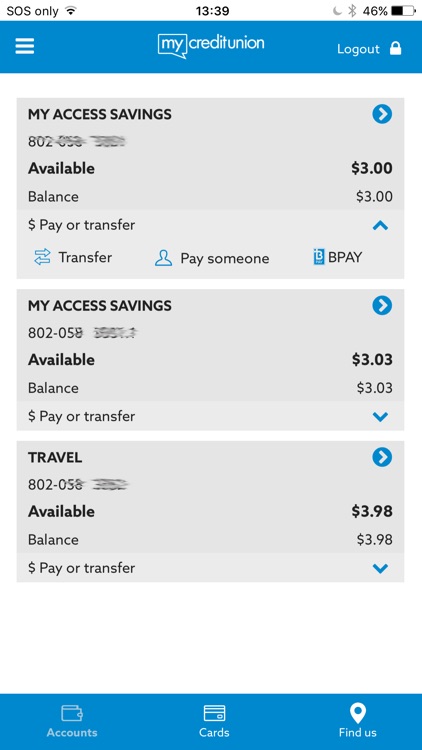This is a detailed screenshot of a digital banking interface. At the top of the screenshot, a blue bar spans horizontally across the screen. On the left side of the blue bar, there is a menu icon represented by three stacked lines. In the center of the bar, the text "My Credit Union" is prominently displayed. On the right side, there is a "Logout" option accompanied by a small white padlock icon symbolizing secure access.

Beneath the blue bar, three distinct gray boxes are aligned vertically, each providing specific account information. 

The first gray box is titled "My Access Savings." It includes details such as "Available Balance" and the options "Money," "Pay," or "Transfer." At the bottom of this box, buttons show options for "Transfer," "Pay Someone," or "BPAY."

The second gray box, also titled "My Access Savings," displays that the "Available Balance" is 303, with an actual balance also stated as 303. It features a "Pay or Transfer" option with a downward-facing arrow, indicating further actions or a dropdown menu.

The third gray box is labeled "Travel" in the top left corner. It details a number, with "Available Balance" and "Pay or Transfer" options below. On the right, it shows the amounts $3.98 and $3.98 again underneath, indicating the available and actual balance respectively.

At the very bottom of the screen, another blue bar provides navigation options with labels "Accounts," "Cards," and "Find Us."

This organized layout allows users to easily manage their finances, with clear options for transferring money, making payments, and accessing important account details.